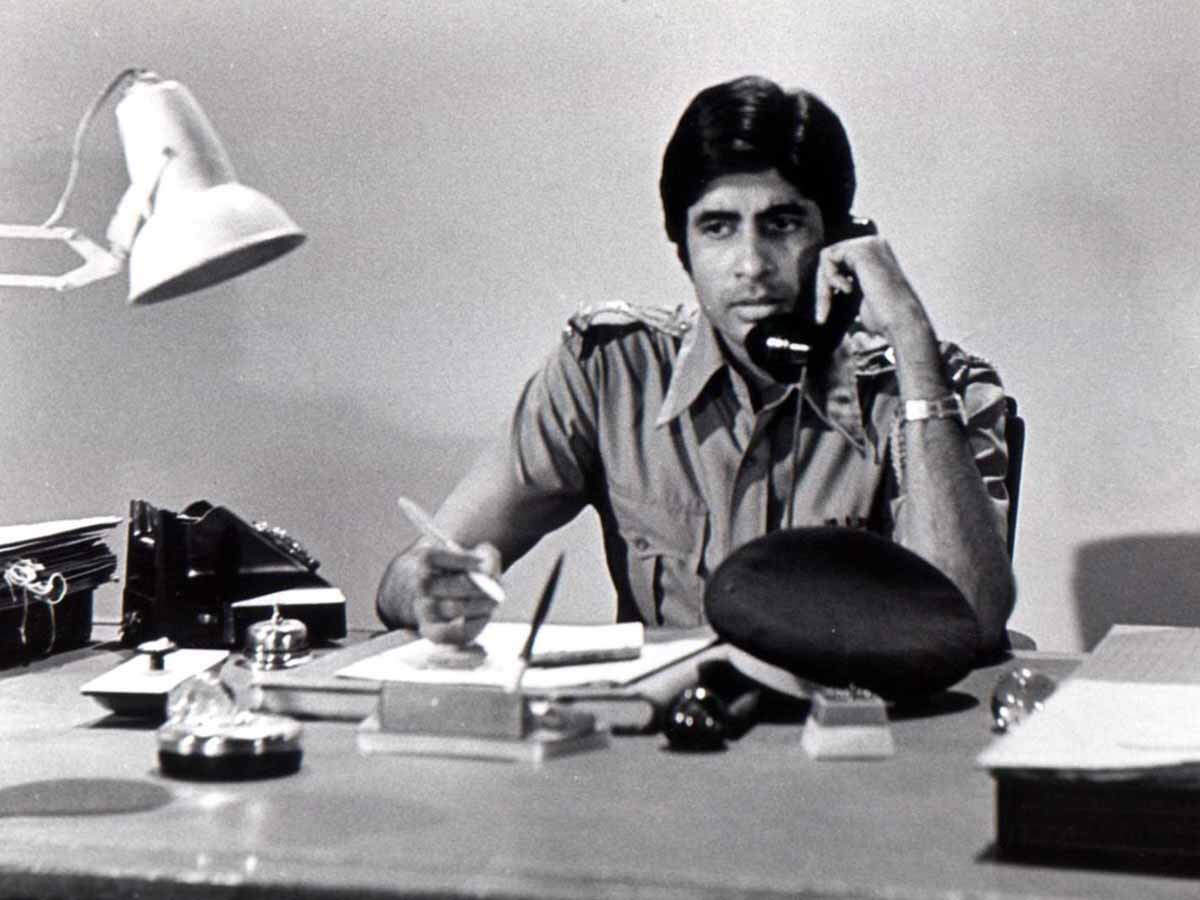This black-and-white photograph appears to be a scene from a movie set, possibly depicting a Mexican police station. The focal point is a man, potentially Hispanic, with neatly groomed short black hair, sitting at a desk. He is attired in a collared button-down military-style uniform with epaulets on the shoulders. On the desk before him, there is a prominent police hat, suggesting his professional role.

The man is engaged in a phone conversation, holding an old rotary phone receiver in his right hand and a pen in his left. A notebook lies open in front of him, and on his wrist, he wears a watch. The cluttered desk is adorned with various office items including paperweights, a lamp with an adjustable arm, a bell, a stack of file folders, and papers indicative of a typical office or police station environment. A plaque is also visible, contributing to the professional setting. The background is nondescript, focusing the attention entirely on the subject and his immediate surroundings.